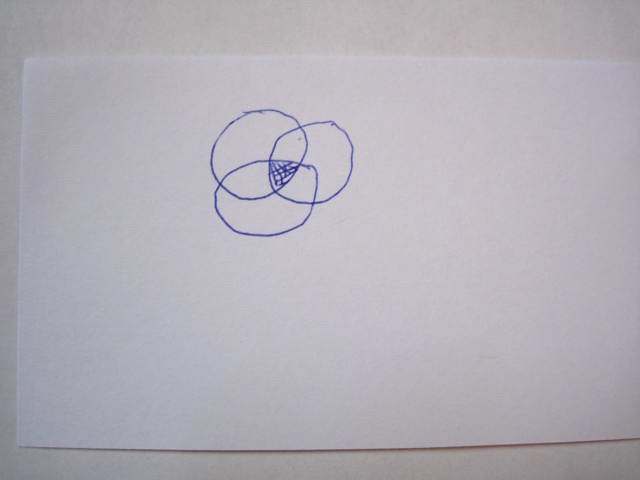A drawing, penned on a rectangular sheet of drawing paper laid horizontally, extends nearly from the far right to the far left within the image frame, leaving only a narrow margin of unoccupied space. The backdrop consists of a solid white wall that seems to be constructed from wood, providing a simple and clean contrast to the artwork.

At the center-left of the drawing, three imperfect circles have been sketched using a blue ballpoint pen. The largest of these circles is positioned at the top left, the smallest rests at the top right, and the widest circle is found at the bottom center. Their edges intersect, creating a central area filled with intricately drawn horizontal and vertical lines that form a grid-like pattern of small squares. The deliberate imperfection and straightforward design lend the drawing an intriguing, handmade quality.